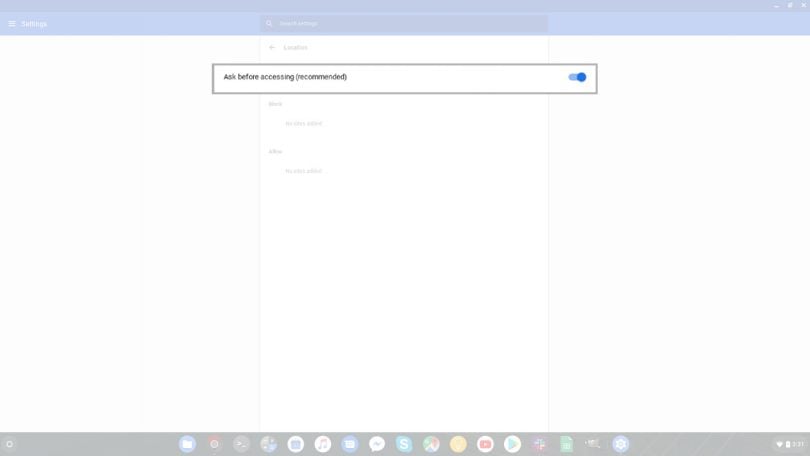The top portion of the image features a long, light blue rectangle. Positioned a few inches below is another rectangle, containing the text "Ask Before Accessing" with "(Recommended)" written in parentheses. On the right side of this rectangle, there is a blue circle. The left side of the rectangle has a lighter blue hue, creating a subtle gradient effect. The bottom section of the image, which appears grayed out, draws less focus but contains a notable element: a long gray bar filled with various circles. 

These circles each contain different icons, including:
- A blue circle with a flag.
- A white circle with a red square and arrow, representing YouTube.
- A blue square with an "S" for Skype.
- A white circle with a blue and pink music note.
- An icon resembling a green battery or piece of paper.
- A blue circle with a white gear icon, representing the Settings app.
- A circle in the center displaying the Google Maps icon.

This collection of icons suggests a navigation or access panel, with each symbol representing a different application or feature.